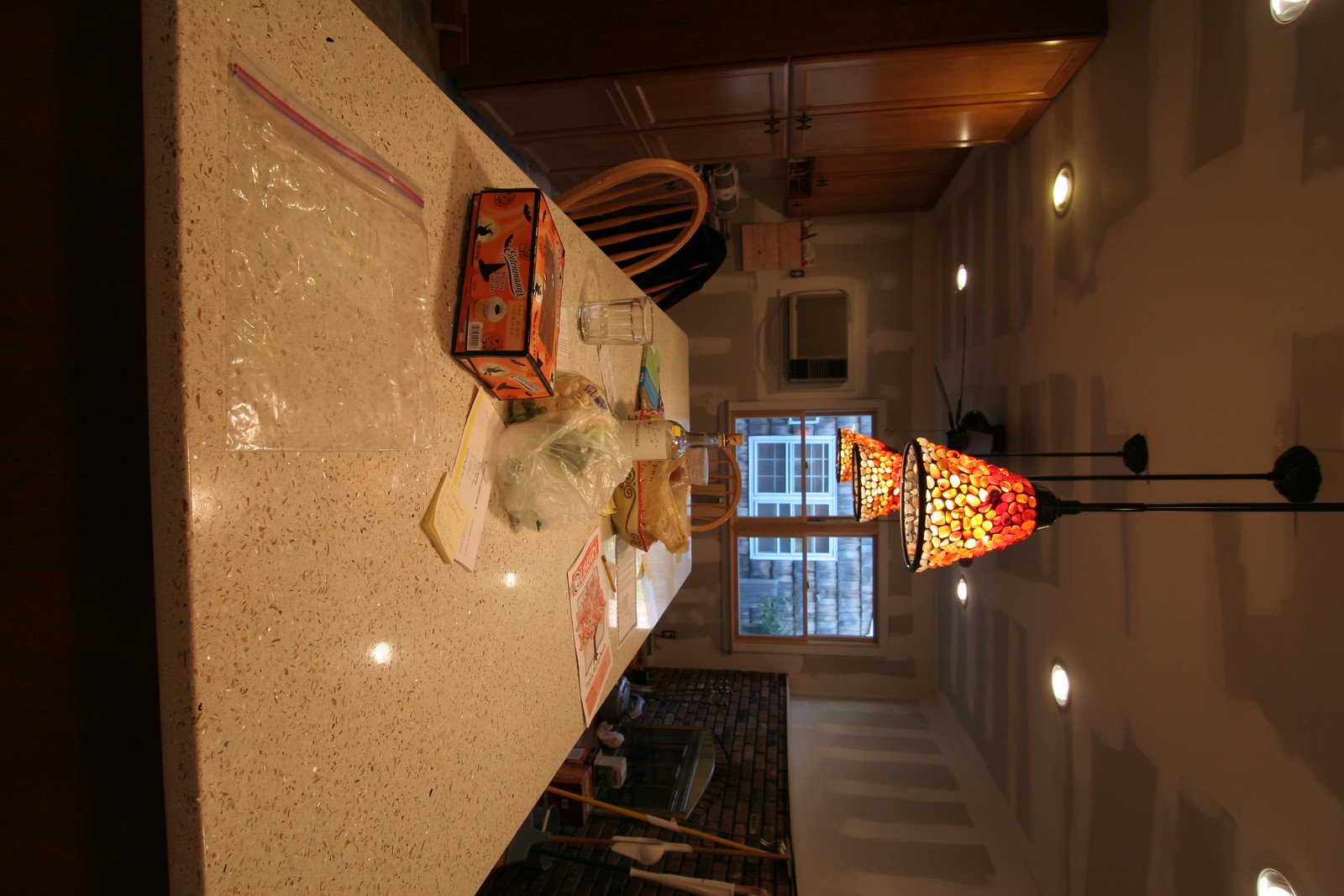The photo is rotated 90 degrees counterclockwise, placing the floor on the left and the ceiling on the right. Dominating the center of the image is a large marble slab, likely serving as a table or kitchen island, cluttered with various items including ziplock baggies, papers, a box, a cup, a basket, and what appears to be a bottle of wine. A plastic bag containing an indistinguishable item is also visible. A single chair is pulled up to the counter, positioned against the backdrop of tall, wooden cabinets. The far wall is unfinished, revealing plaster marks and patches. To the right, a double-paned window, framed in dark wood and accompanied by an air conditioner, hints at ongoing renovations. The ceiling shows lighting fixtures and three large lamps in red and yellow hues. Below, a section of the wall exposes brickwork with numerous objects propped against it, adding to the sense of disarray and incompleteness in the room.